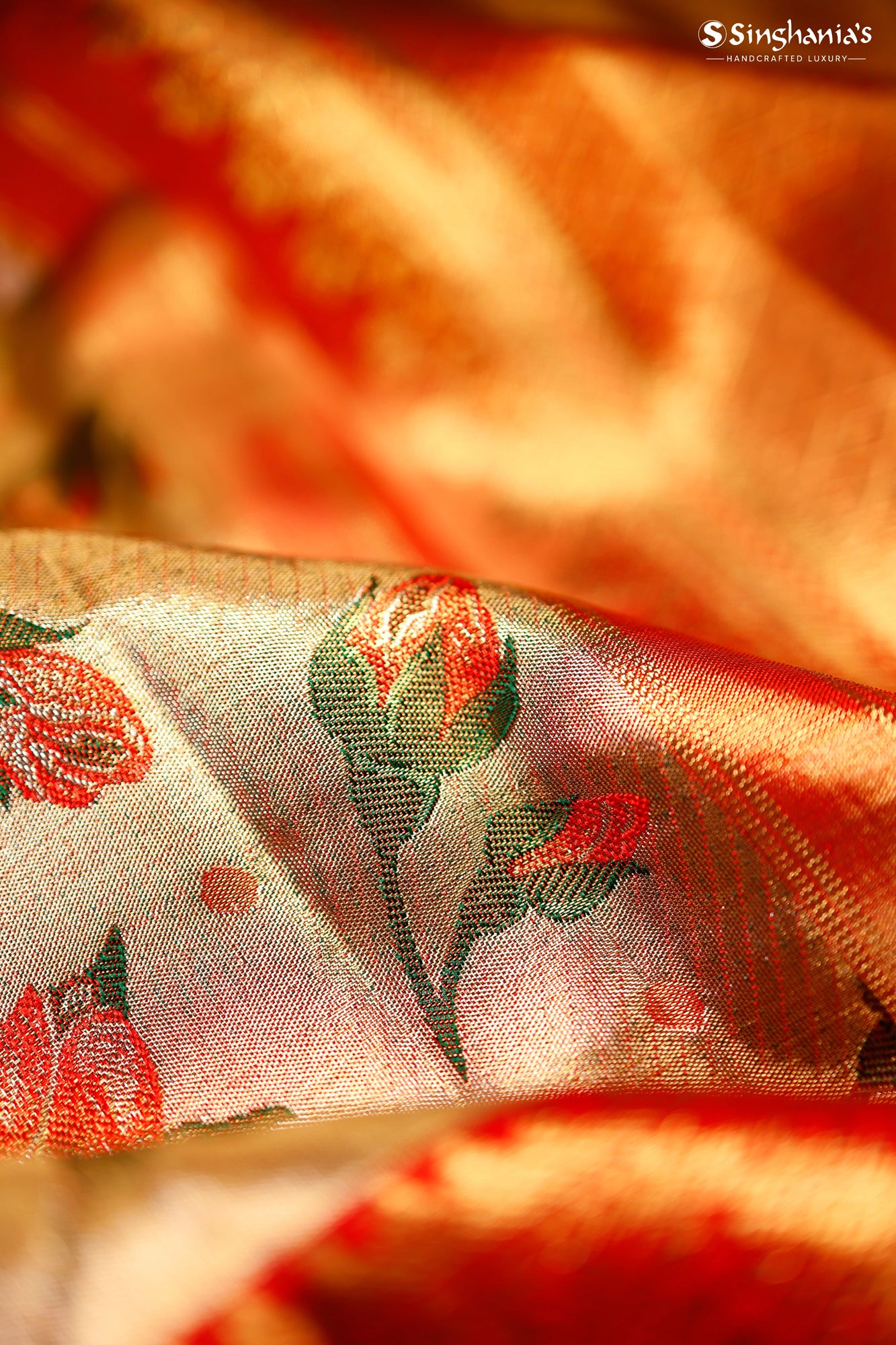This vertical rectangular image presents an up-close photograph of a luxurious, handcrafted fabric, likely silk. The main focus of the image is a vibrant, detailed pattern set against a background of out-of-focus red, yellow, and orange fabric. Dominating the center of the frame is an intricately embroidered section, featuring a series of red flowers with green stems and leaves. The light yellow background of the fabric enhances the colors, making the red flowers especially vivid. In the upper right corner, the text "S. Shingania's Handcrafted Luxury" is displayed in white font. The out-of-focus areas in both the background and foreground of the image reinforce the texture and richness of the silk material.